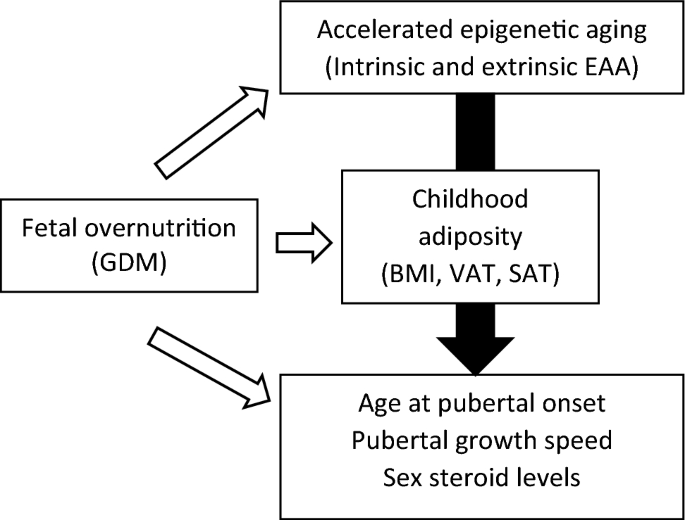The image is a detailed black-and-white flowchart that diagrams the effects of fetal overnutrition, designated with the abbreviation GDM. The central rectangle labeled "fetal overnutrition (GDM)" on the left side of the chart has three arrows originating from it, each pointing to distinct subsequent outcomes illustrated in separate rectangles. 

The top arrow directs attention to a rectangle labeled "accelerated epigenetic aging," with an annotation "(intrinsic and extrinsic EAA)" underneath. Another arrow from this rectangle proceeds downward, linking it to the middle rectangle. This middle rectangle, also directly connected by its own arrow from the initial "fetal overnutrition" box, is labeled "childhood adiposity," with the specific measures "BMI, VAT, SAT" in parentheses. 

The final, bottom arrow from the "fetal overnutrition" rectangle points to a rectangle captioned "age at pubertal onset," further detailing "pubertal growth speed" and "sex steroid levels." Additionally, a connecting black arrow from "accelerated epigenetic aging" also points downwards, emphasizing the linkage to "age at pubertal onset." The flowchart visually represents the interconnected biological and medical impacts of fetal overnutrition as outlined in scientific or medical literature.